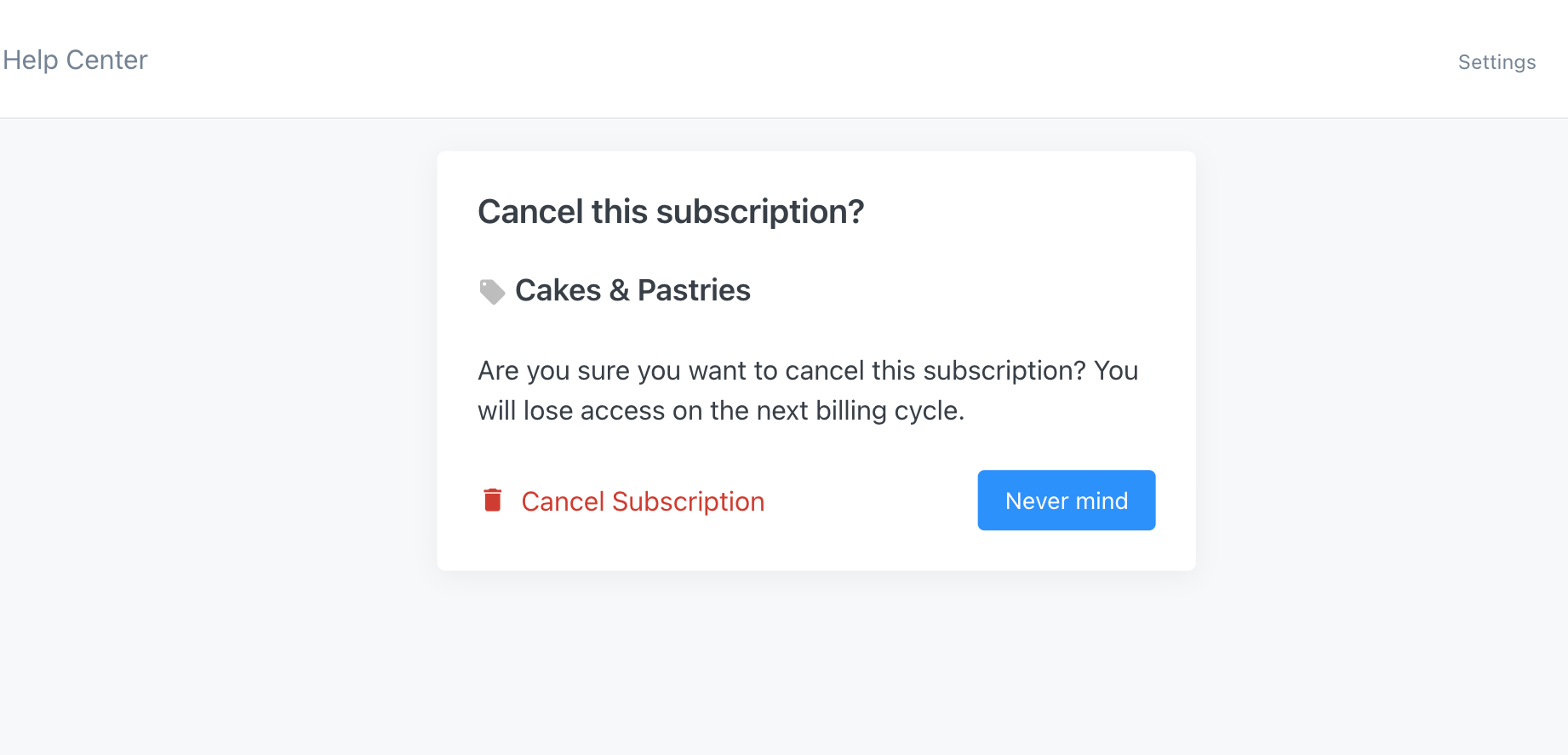This image depicts a webpage with a predominantly horizontal layout. The top left corner features the "Help Center," written in black text. In the top right corner, there is a smaller black text caption for "Settings." These elements are set against a white background, devoid of any color.

Directly beneath this header section, the background transitions to a light blue hue. Central to the image is a prominent white dialog box. This dialog box presents a confirmation message, specifically titled "Cancel this subscription?" Below this title, there is an icon resembling a price tag, adjacent to the text "Cakes and Pastries."

The dialog continues with a warning statement: "Are you sure you want to cancel this subscription? You will lose access on the next billing cycle." Following this is a red icon depicting a garbage can, next to the words "Cancel Subscription." This option indicates the action to confirm the cancellation.

At the bottom corners of the dialog box are two blue buttons. The button on the left displays the word "Nevermind" in white text, as does the identical button on the right. There is no other text or significant detail present in the image.